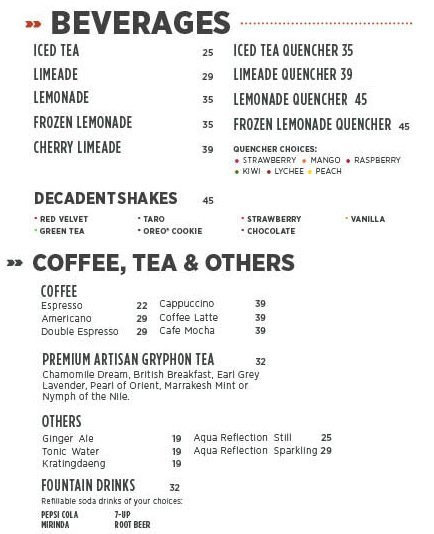This image shows a scan or picture of a menu featuring the beverages section in bold black text at the top, with a red dot horizontal separator underneath. The beverages are organized into two columns. Listed first are the prices for iced tea (25), limeade (29), lemonade (35), frozen lemonade (35), and cherry limeade (39). This is followed by a variety of iced tea and limeade quenchers, along with their corresponding prices.

Below this, there is a section for decadent shakes, each priced at 45, featuring flavors such as red velvet, green tea, taro, Oreo cookie, strawberry, chocolate, and vanilla.

Further down, there is another major section titled "Coffee, Tea, and Others." The coffee subsection includes options like espresso, americano, double espresso, cappuccino, latte, and mocha. The tea offerings include premium artisan griffin tea, chamomile dream, British breakfast, Earl Grey, lavender, pearl of orient, marquish mint, and nymph of the Nile.

Finally, the "Others" subsection lists beverages such as ginger ale (19), tonic water (19), aqua reflection still, aqua reflection sparkling, and various fountain drinks including Pepsi, Mirinda, 7Up, and root beer, with refillable soda drinks priced at 32.